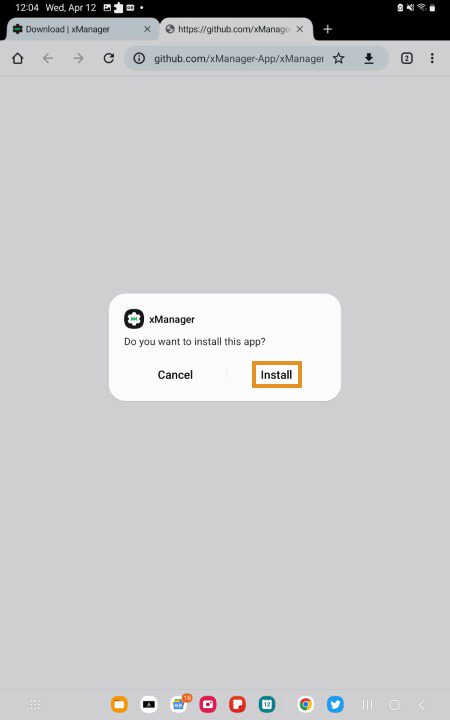This vertical rectangular image features a predominantly black header at the top. In the top left corner, in white font, it displays the time "12:04" with the day "WED" (short for Wednesday) and the date "APR 12" (for April 12th). In the top right corner, there are tiny white icons typically representing notifications and system status indicators.

Beneath the header, the screen is divided into two dark gray tabs. The first tab displays "Download X manager" with the "X" in lowercase and "Manager" capitalized. To the left of the text is a small icon suggesting a download symbol. The second tab contains a web address formatted as "https://github.com/Xmanage," which also has a small icon to its left. There is an additional tab represented by a plus "+" sign, which is not opened.

The main section of the screen highlights this web address in the browser's search bar. Dominating the center of this gray interface is a white pop-up window. In black font, it asks, "X manager: Do you want to install this app?" Below this prompt, there are two options: "Cancel," written in black, and "Install," highlighted with a gold ring around it.

At the bottom of the image, a row of various colorful icons is noticeable, likely representing different apps or functionalities on the device.